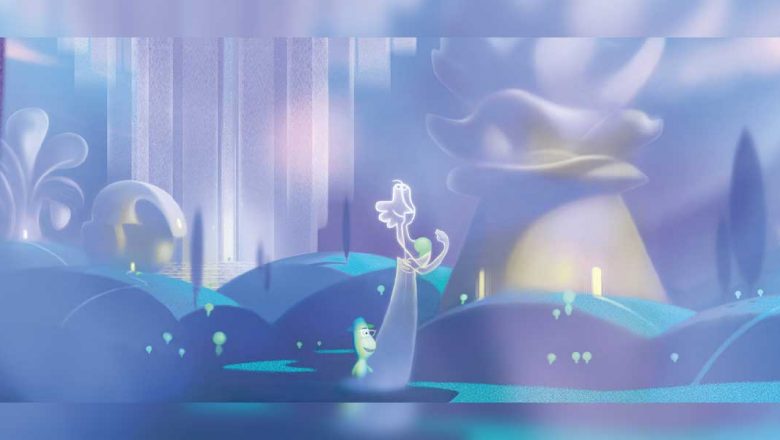The image is a rectangular, fantasy-style illustration predominantly in various shades of blue, ranging from sky blue to darker blue, with an ethereal, white overcast or fog lending it a dreamlike quality. In the background, swirls of lavender, pink, blue, gray, silver, and golden bronze hues add depth and complexity. A notable feature is the band at the bottom, reflecting the scene above, possibly resembling water. Central to the image is a tall, wispy, translucent figure, standing with arms raised towards the sky, wearing a long bluish dress outlined vividly in white, giving it an angelic appearance. To the right, there are rolling turquoise-colored hills and a series of dark blue to sky blue hills, with a hovering white light area above them. The left side showcases white lines that could be beams of light or a waterfall, enhancing the mystical ambiance. Among the surreal landscape are distinctly illustrated characters: a luminous figure clad in a white dress, possibly a ghost, holding something green; and a shorter, whimsical green figure with a jellybean face, wearing a turquoise top hat and orange glasses. Nearby, a purple tree stands tall, accompanied by Italian cypress-like trees. The overall scene is reminiscent of a whimsical Disney movie with its enchanted and animated characters.